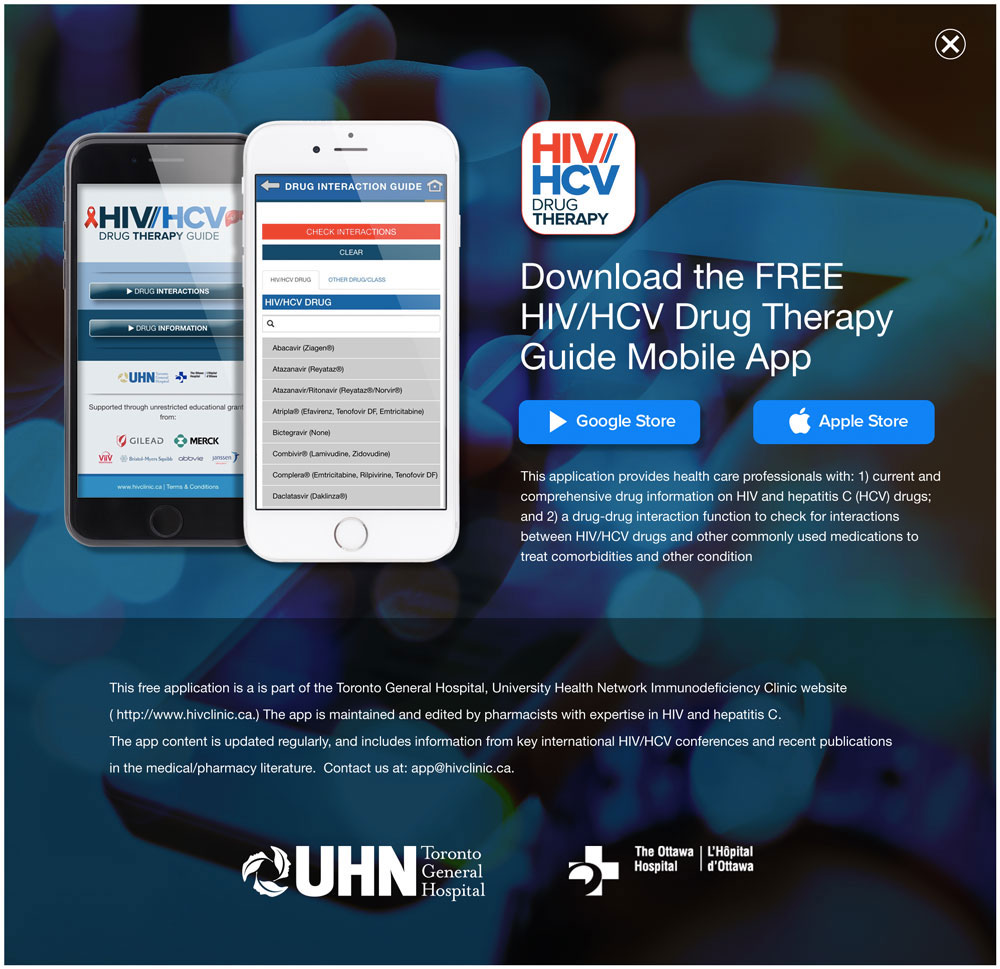This image features a detailed display primarily focused on a map set within a webpage. On the left side of the image, a hand is visible in the background. To the right of the hand, a smartphone is tilted on its side.

In the top right corner of the image, there is a circular icon with an 'X' in it, indicating it is likely a part of a webpage interface. Below this, two smartphones are prominently displayed. 

The left phone, with a black case, shows a screen titled "HIV-HCV Drug Therapy Guide." The right phone, in a white case, displays "Drug Interaction Guide." Beside these phones is a box with a white background containing text.

In this box, the words "HIV-HCV Drug Therapy" are at the top, followed by the text "Download the free HIV-HCV Drug Therapy Guide" in white lettering. Below, there are two blue buttons labeled "Google Store" and "Apple Store." Under these buttons, white text provides a description of the application:

"This application provides healthcare professionals with:
1. Current and comprehensive drug information on HIV and HCV drugs.
2. The drug-drug interaction function to check for interaction between HIV, HCV drugs, and other commonly used medications."

The text concludes with "More readings" and mentions additional conditions treated by the application.